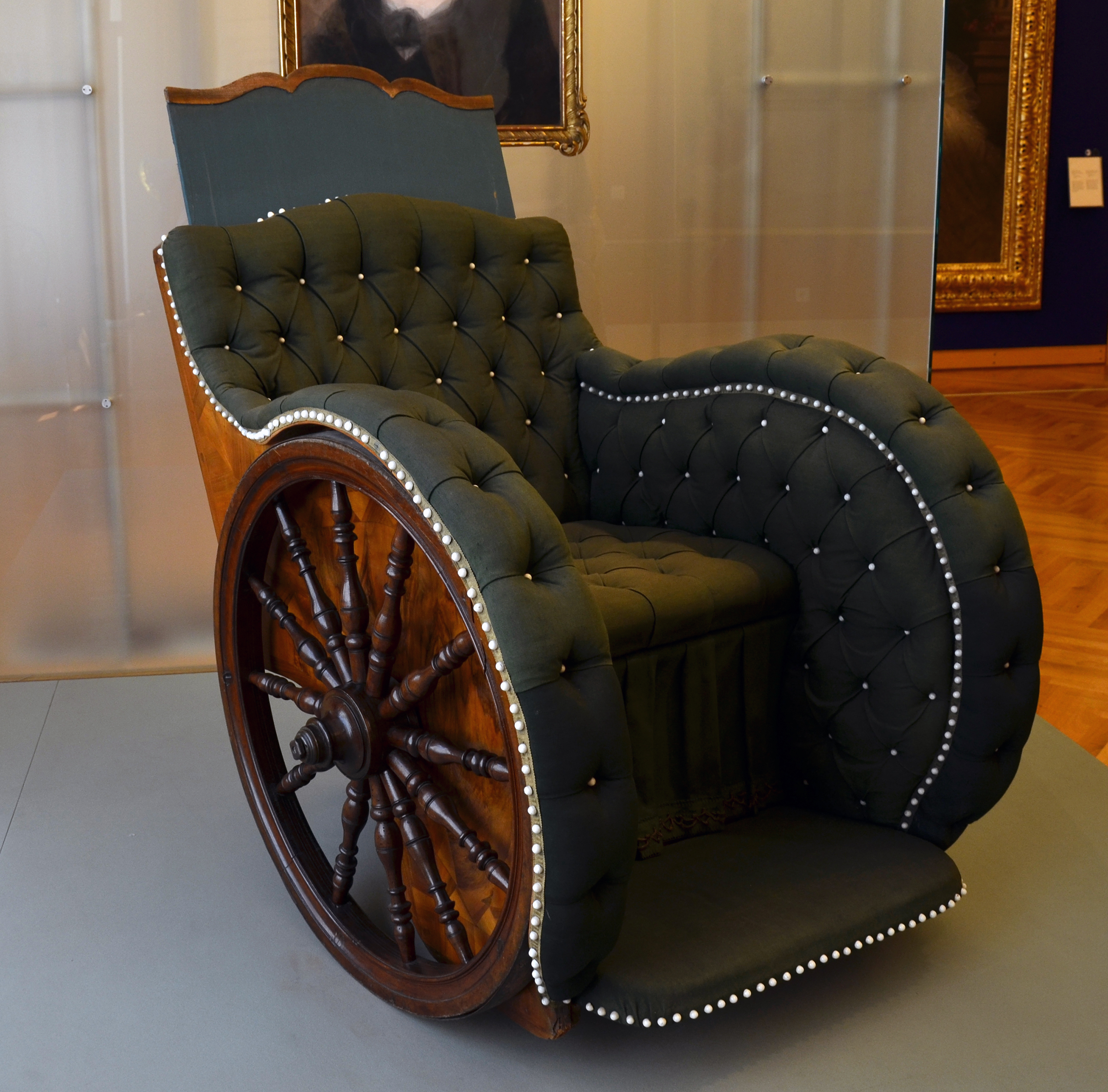In this photograph, an ornate antique wheelchair is prominently displayed in what appears to be a museum setting. The wheelchair is positioned on a gray floor, with a semi-opaque wall behind it. A faint image of a person in a suit is visible through this wall, though the face is obscured. Further back, the flooring transitions to parquet, leading to a large, gilded frame encasing an elegant painting. A piece of paper is taped to the wall near this artwork.

The wheelchair itself is a stunning example of craftsmanship. It features oversized wooden wheels, reminiscent of a ship's wheel, likely crafted from walnut. The seat of the wheelchair is upholstered in a luxurious green quilted fabric, adorned with buttons in each quilted segment. A high headboard and pearl decorations embellish the sides, enhancing its opulent appearance. The entire design exudes comfort and sophistication, with plush, thick cushions inviting anyone to sit.